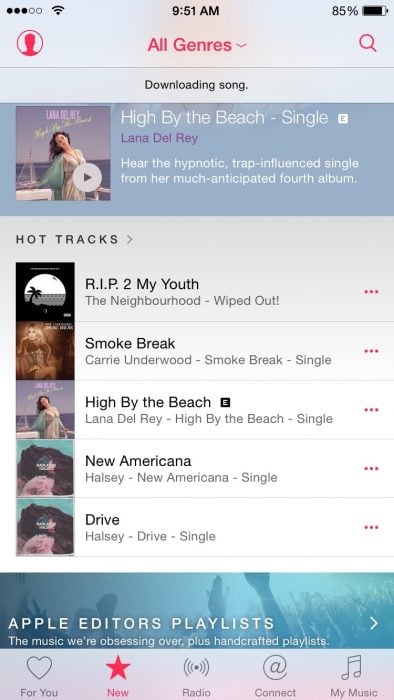A digital screenshot centered on music displays the time, 9:51 AM, at the top. Featured prominently is the song "High by the Beach" by Lana Del Rey. This hypnotic, trap-influenced single is from her much-anticipated fourth album. Beside the title, there is an image of Lana Del Rey standing on a balcony near the water, her head tilted back, adorned in a shimmering silver-colored dress, appearing to be around 37 years old.

Further down, under the section titled "Hot Tracks," the song "R.I.P. to My Youth" by The Neighbourhood from their album "Wiped Out!" is listed, accompanied by an image of a palm tree.

Beneath this, "Smoke Break" by Carrie Underwood is mentioned, characterized as a single. To the left of the title, there's a picture of Carrie Underwood, a white woman with blonde hair, who appears to be around 40 years old. She is sitting with her legs crossed, wearing shorts.